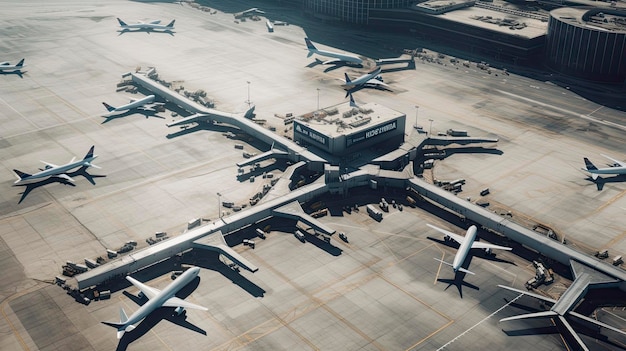This detailed aerial photograph captures a bustling airport concourse on a sunlit day. The concourse is laid out in a plus sign configuration, where three arms are fully extended while the fourth is not. Surrounding the concourse, there are numerous passenger aircraft, with approximately ten commercial jets of various sizes—predominantly two-engine jets—visible throughout the scene. 

In the upper right of the image, several large buildings are prominent, with one particularly notable for its height, spanning a few floors. While the specific functions and labels of these buildings are unclear, the central terminal features some indistinguishable writing. Aircraft are seen docking at the concourses, taxiing between gates, and moving toward or away from the runways. 

The concourses themselves extend from the central terminal in three primary directions: one arm stretches to the top left, another to the bottom left, and the third to the bottom right. The overall activity paints a picture of a fairly busy but orderly airport environment.